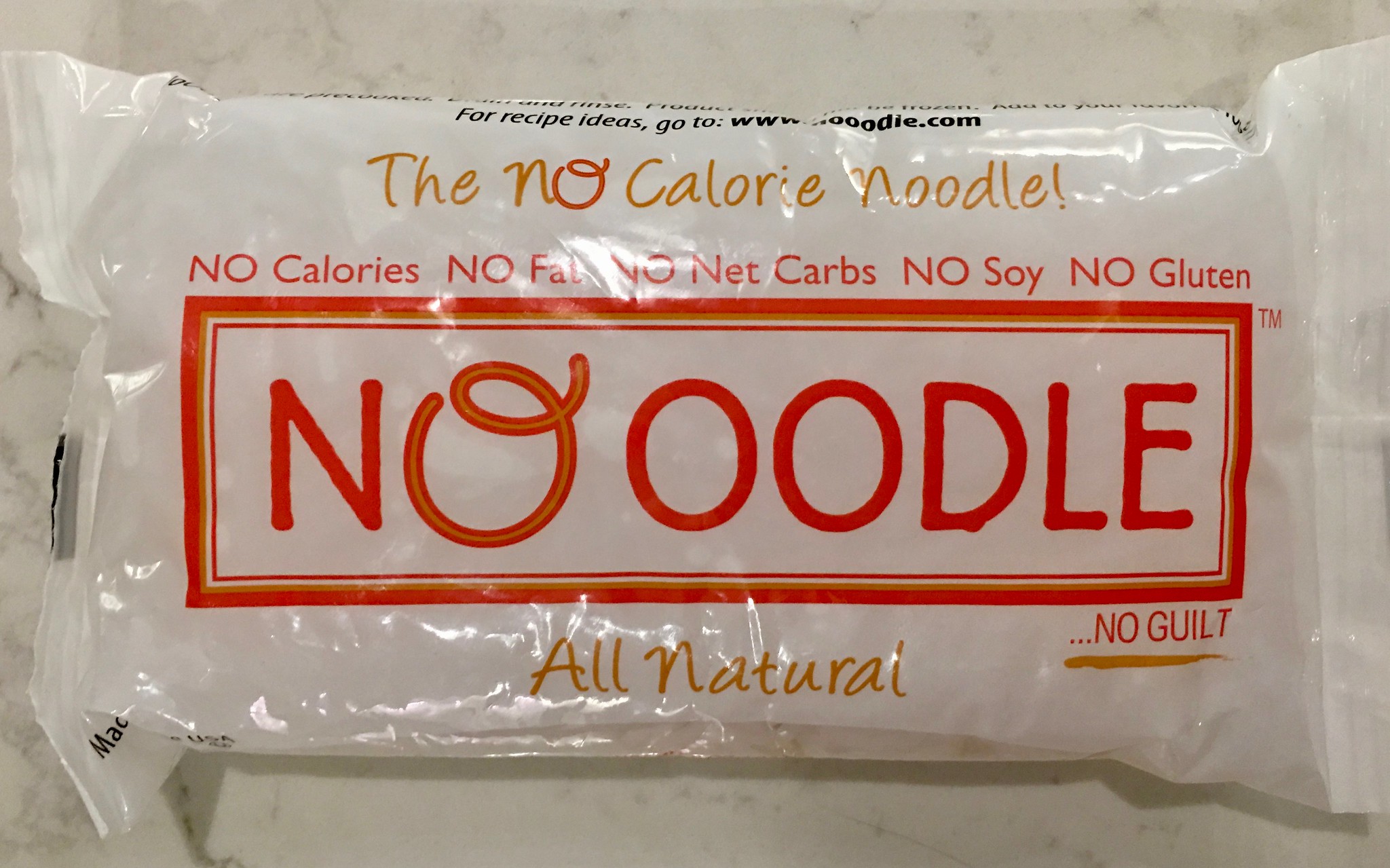The image features a translucent white package prominently displaying the branding and product information for "Noodle," stylized as "NOOOODLE" in large, bold red letters centered within a rectangular red sign. Just below this sign, there is a yellow label stating "All Natural." In the bottom right-hand corner of the red sign, the words "No Guilt" are written in red letters. Positioned above the rectangular sign are a series of health claims in red text: "No Calories, No Fat, No Net Carbs, No Soy, No Gluten." At the very top of the package, in slightly larger yellow lettering with the exception of a red 'O,' it reads "The No Calorie Noodle."